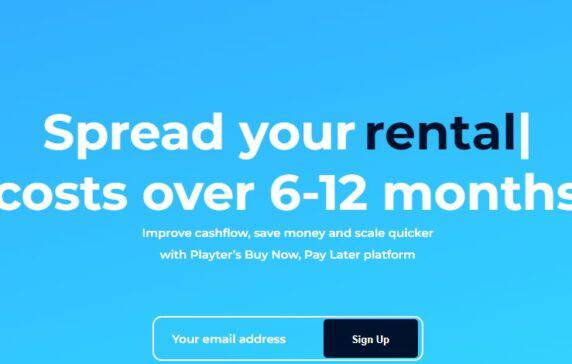### Detailed Caption

The image is a screenshot of a web page that has a predominantly light sky-blue background. However, the image quality is compromised due to significant JPEG artifacting, especially around the text and other elements.

At the top of the image, there is a heading in white text that reads, "Spread your rental costs over 6-12 months." The word "rental" is distinctly highlighted in a very dark blue color. Interestingly, there is an extraneous white vertical line, also known as a pipe (|), placed at the end of the word "rental" that doesn't appear to serve any specific purpose.

Below this main heading, there is a subheading in white text that states, "Improve cash flow, save money, and scale quicker with Plater's Buy Now, Pay Later platform." This text aims to highlight the benefits of the payment service being promoted.

Further down, there is a thin white rectangular box which has the placeholder text "Your e-mail address" inside it. To the right of this box, there is a dark navy blue button, almost black, with the words "Sign Up and Sign In" written in stark white letters.

Overall, the combination of light sky blue, dark navy blue, and white text aims to create a visually appealing interface, though the heavy JPEG artifacting significantly detracts from the clarity and sharpness of the image.